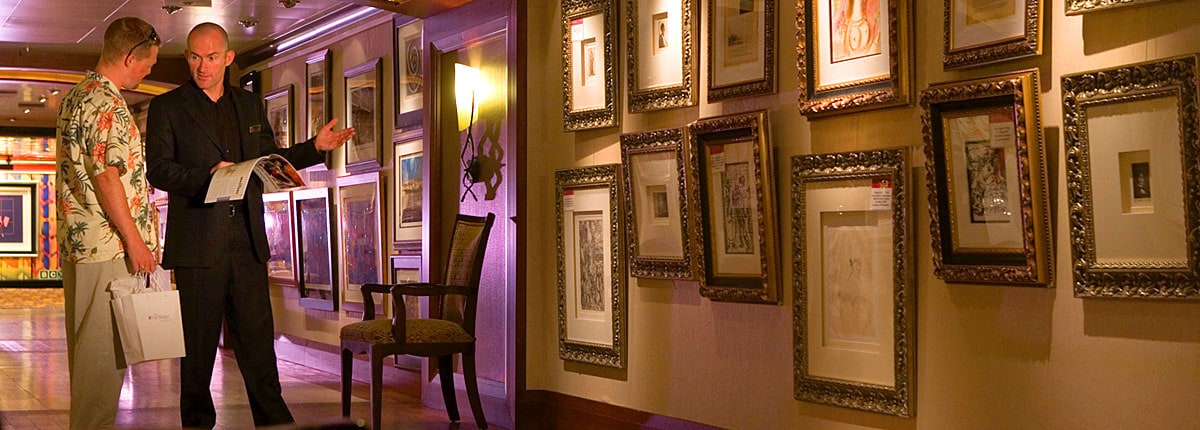In this detailed scene set in an elegant art gallery, possibly aboard a cruise ship, two men are engaged in an animated conversation amidst an array of framed artworks displayed closely along the tan-colored walls of the corridor. Price tags are visible beneath each piece, underscoring that all the artworks are for sale. The customer, dressed casually in a Hawaiian shirt and khaki pants with sunglasses perched on his head, holds a white shopping bag, likely containing items purchased from another store. On the other hand, the gallery worker, clad in a black jacket with a name tag and black pants, holds a brochure or program and appears to be enthusiastically explaining the details of a particular piece of art. Between two exhibits, a brown chair with white cushions and a light sconce above adds to the upscale decor of the setting, enhancing the sophisticated atmosphere of this art-filled space.